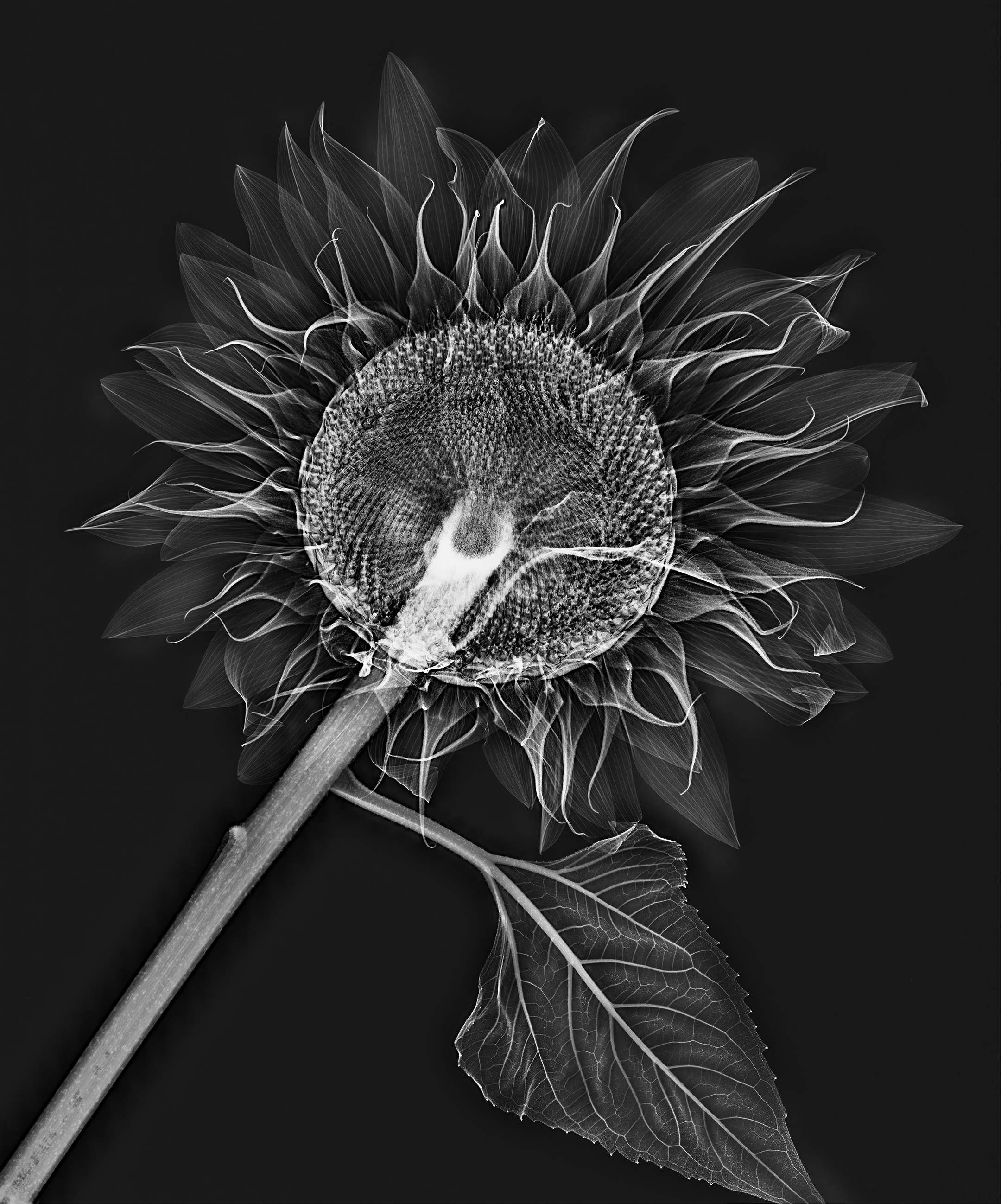The image appears to be an x-ray of a flower, showcasing intricate details in black and white. Set against a solid black background, the flower itself stands out in varying shades of gray and white. The main focus is on a central bulb-like structure surrounded by delicate, ethereal petals that give a fiery impression. Stretching from the lower left corner towards the upper right, a lighter-colored stem supports the flower, with a noticeable leaf protruding from the right side just below the central bulb. The petals become gradually more gray as they extend outward, creating a delicate, almost translucent look. The unique portrayal resembles a dandelion or possibly a sunflower, capturing what could be an artistic interpretation via an x-ray-like technique.